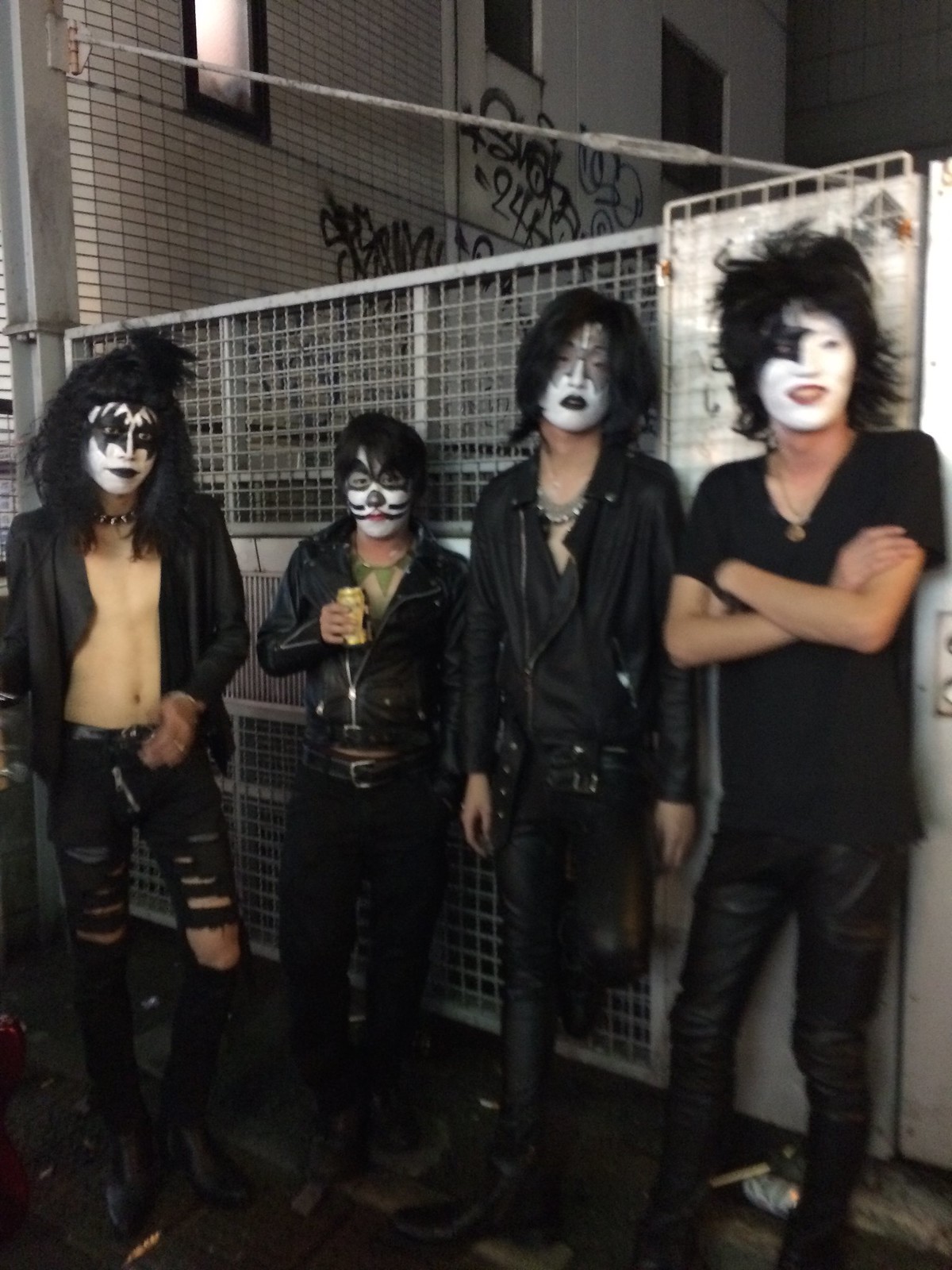This outdoor photograph, likely taken in Japan given the architecture, captures four young, thin Asian men in their early 20s posing in front of a tall, white brick-tile building with frosted windows and black graffiti. Their attire and makeup resemble the iconic rock band KISS, featuring black and white face paint with distinct designs. Each man is adorned in tight-fitting black clothing, including black jeans or leather trousers, leather jackets, and accessories like necklaces. The scene appears to be set on a dimly lit street and slightly blurs out of focus on the right side. The man on the far left sports tight, torn black jeans and a black jacket with no shirt. The middle-left individual, holding a drink in his right hand, has green triangles around his neck and a feline-inspired face paint. The middle-right person, possibly looking at the photographer, wears a baggier black jacket with his left leg lifted. Lastly, the man on the far right, who is slightly out of focus and smiling, features a star over his right eye and has his arms crossed. They all stand in front of a metal gate, exuding a strong rock and roll vibe.